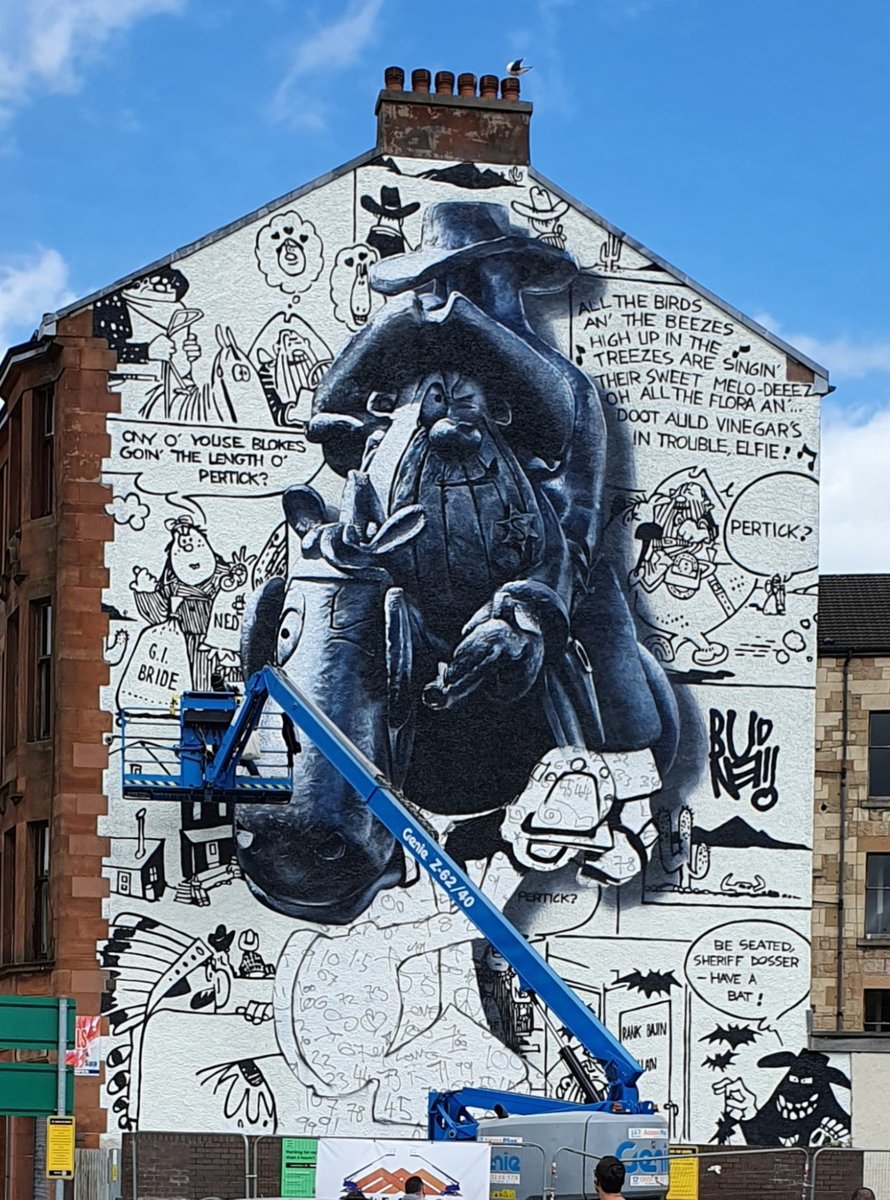The image depicts a color photograph of the side of a brick building that has been entirely painted white. Covering this white facade are intricate black cartoon illustrations reminiscent of old newspaper comics. Central to the artwork, a rugged character wearing a hat, who looks notably depressed, holds a gun. There’s also an imposing figure with a beard holding a sheriff’s badge, accompanied by another man who seems to be hugging him.

Above these characters, whimsical text bubbles display intriguing phrases like, "Onios, ewes, blokes, go in the length of Pirtik," and "All the birds and the beeses high up in the treeses are singing their sweet melodieses." A melancholic figure holds a bag labeled "GI Bride," while in the bottom right, a thief is captured in the moment with a bubble overhead that reads, "Be seated Sheriff, doze or have a bath."

Adding to the dynamic scene, a blue crane with someone in the basket is actively painting the mural against the backdrop of a clear, blue sky dotted with white clouds.